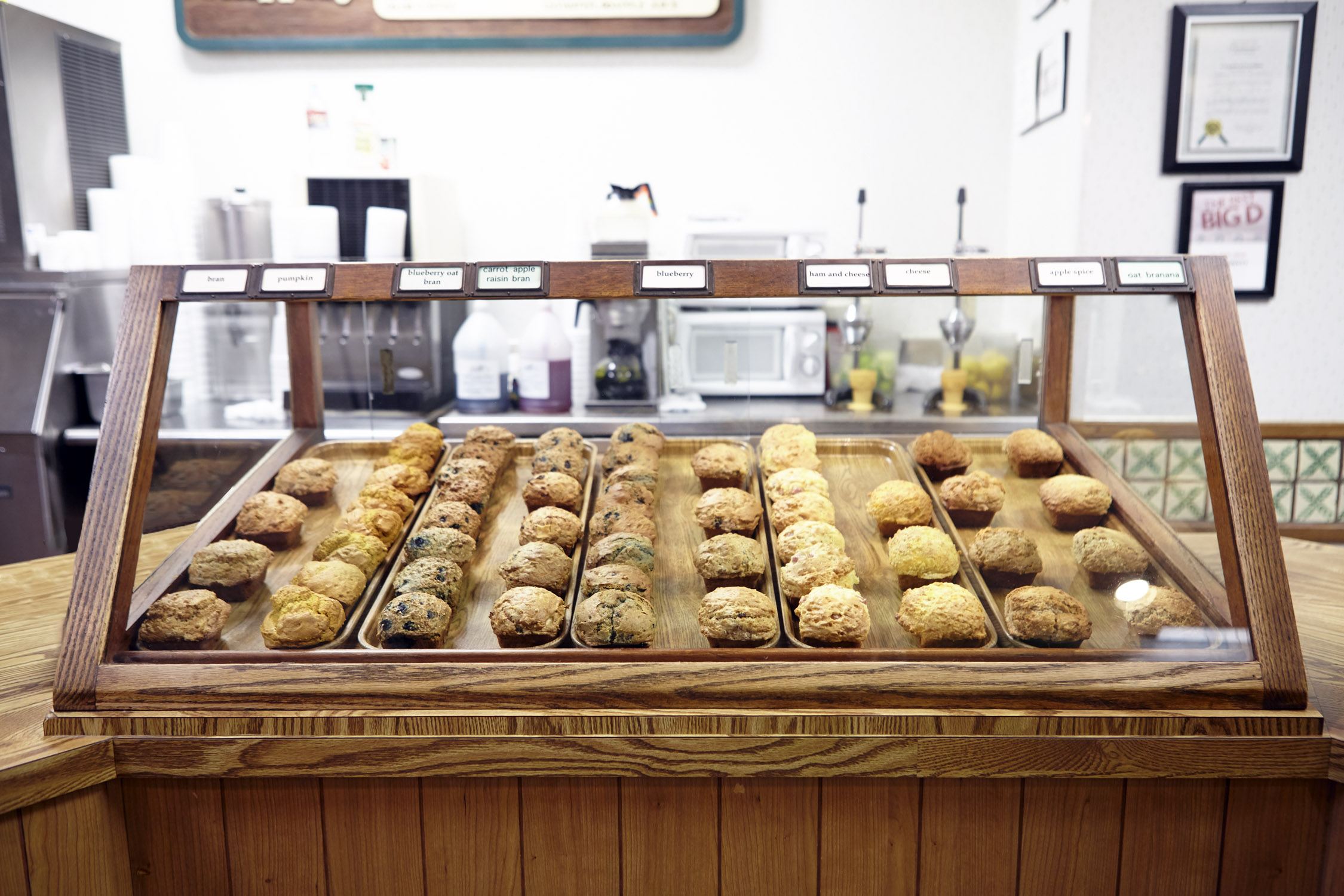This rectangular image, wider than it is tall, captures a detailed scene of a bakery display inside a pastry shop. Central to the image is a wooden counter with intricately paneled wood, topped by a triangular glass pastry case, allowing a clear view of multiple rows of assorted pastries. Organized neatly in five rectangular wooden trays, the pastries appear to be muffins and scones, some labeled with flavors such as pumpkin, blueberry, oat bran, carrot apple, raisin bran, ham and cheese, apple spice, and cheese – though not all labels are legible. The pastries themselves range in color from rich browns to creamy tans. Behind the display, the shop's background reveals a prep area with white walls, stacked cups, a coffee machine, a small oven, and a microwave, along with a few lemons and indistinct signs, lending a cozy, bustling atmosphere to the scene.